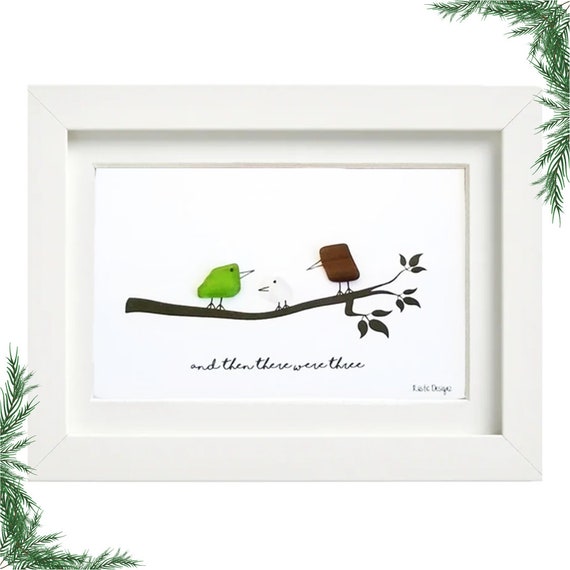The image depicts a simple, yet charming framed drawing. The setting includes a white frame with a white mat, and the background around the frame features evergreen branches subtly peeking in from the top left and bottom right corners, adding a touch of nature. Inside the frame, against a white backdrop, is a delicate illustration of a tree branch with three small branches, each adorned with three pointed leaves. Perched on the branch are three abstract birds: a green bird with a black eye and beak and a rounded bottom resembling a square, a subtly visible white bird with just its eye and beak discernable, and a larger brown bird also appearing square-shaped. The green bird faces left, while the white and brown birds look towards it, as if in conversation. Below the branch, in cursive, the text reads "and then there were three." There's a small, nearly illegible signature and design mark in the left-hand corner, completing the artwork's serene and minimalist aesthetic.